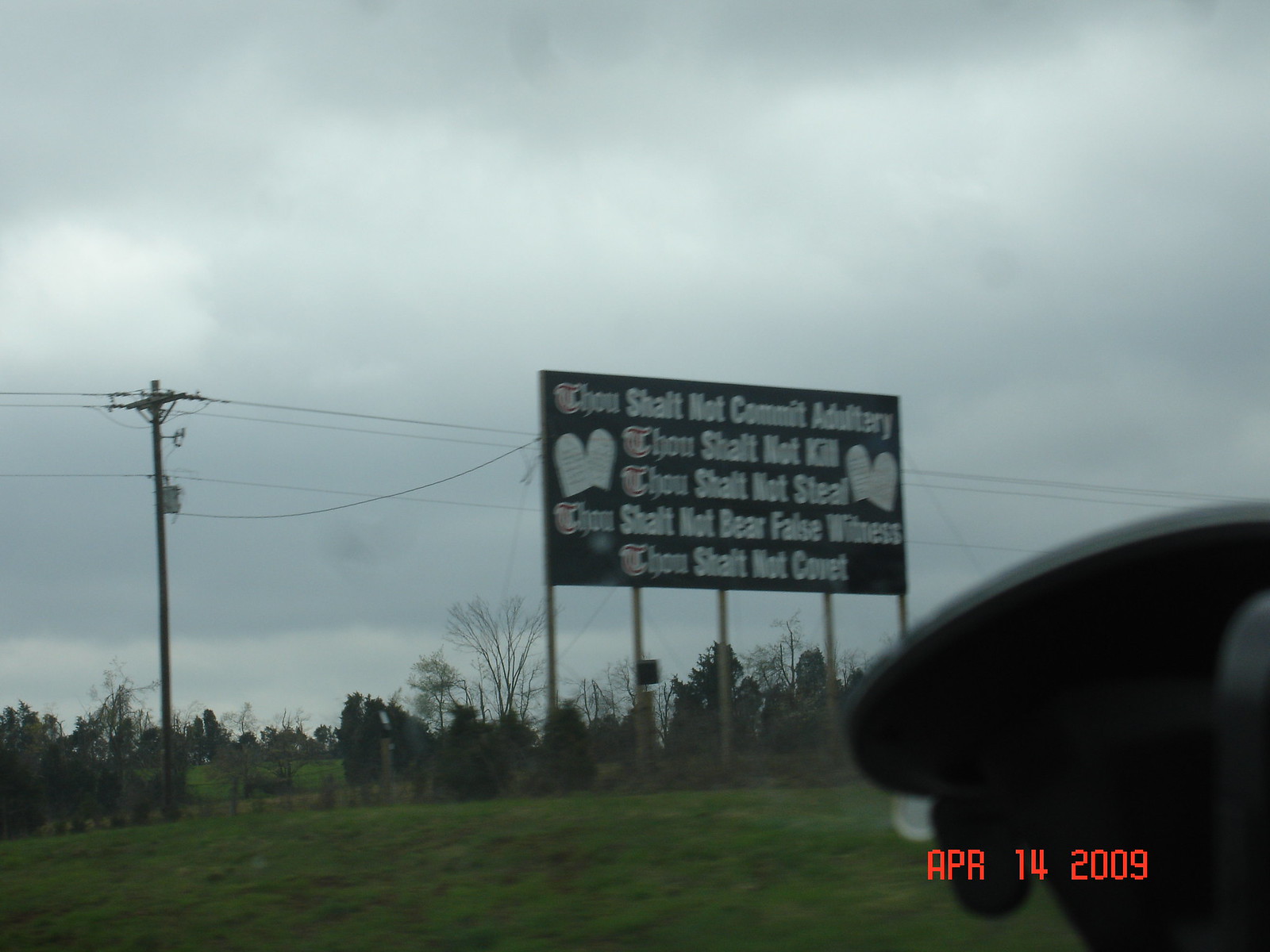The photograph captures a dark evening scene featuring the bottom part of an image with green grass. In the lower right-hand corner, digital-style red lettering displays the date "April 14, 2009." Above the grass, a dark tree line is visible, featuring relatively small trees. On the left side of the image, a utility pole with multiple wires stands against a gray, evening sky.

Dominating the center of the image is a large, dark-background, four-legged billboard-style sign, mounted on five wooden poles. The sign bears white writing stating the following commandments: "Thou shalt not commit adultery, thou shalt not kill, thou shalt not steal, thou shalt not bear false witness, thou shalt not covet." On either side of the sign, there appear to be two small, white tombstone-shaped objects.

Parallel to the sign are visible electricity cables, and a small wooden fence separates two fields in the background. The cloudy sky and the additional dark green bushes add to the somber atmosphere. In the bottom right corner, part of the image is obscured by an indistinguishable, black, blurry, semi-circular object behind the red date font.